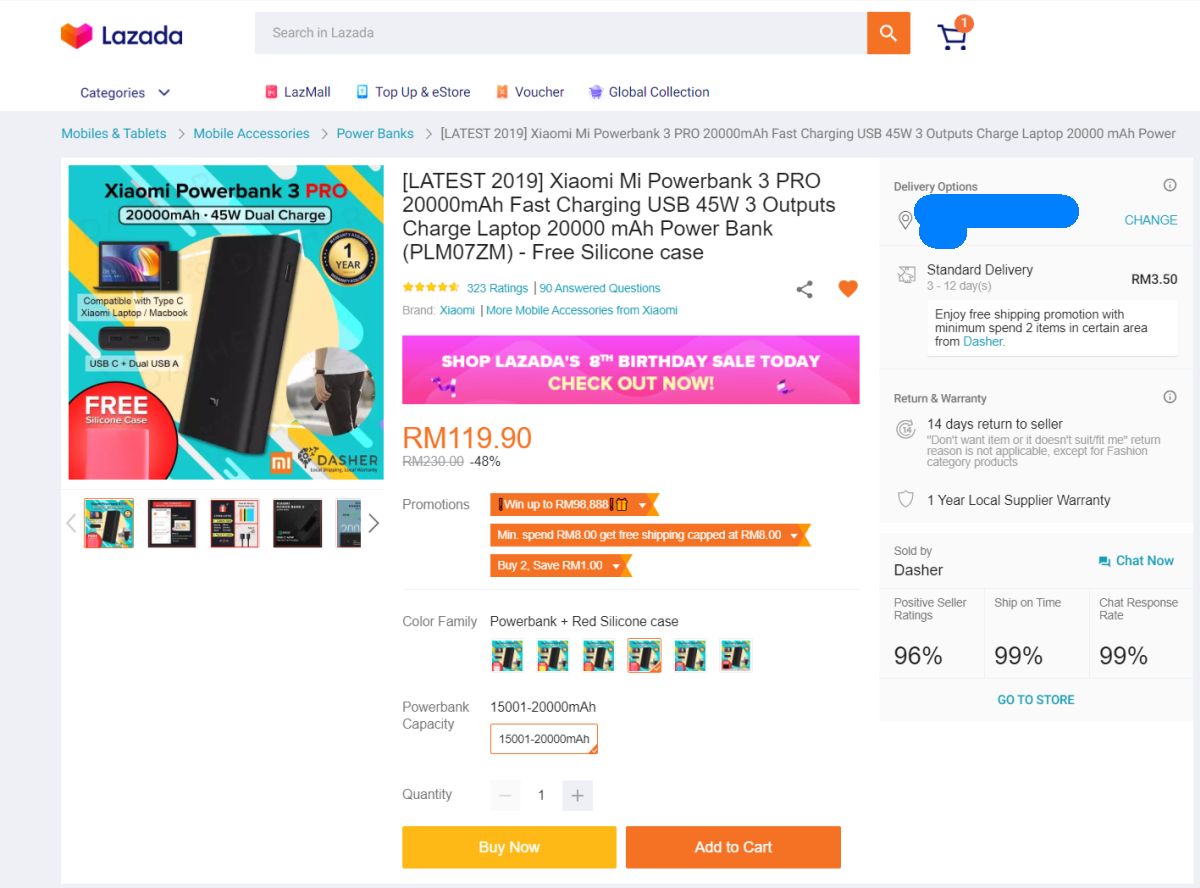Screenshot of Lazada Website Featuring Xeomia Power Bank 3 Pro:

The screenshot captures the Lazada shopping website, displaying a prominent advertisement for the Xeomia Power Bank 3 Pro. At the top of the screenshot, there is a heart icon followed by the word "Lazada." Below this, a search bar is positioned next to a shopping cart icon that shows a quantity of one item.

The primary advertisement is vibrant and showcases a sleek, black Xeomia Power Bank 3 Pro. The ad includes small images of a MacBook and a USB-C charger, emphasizing the compatibility of the power bank with these devices. Accompanying the product image is a note mentioning a complimentary silicone case and a circular icon indicating a one-year warranty.

To the right of the product image, text details the product description, marking it as the "Latest 2019 Xeomia MI Power Bank 3 Pro." User engagement metrics show 323 ratings and 90 answered questions concerning the product.

A notable pink rectangular box within the ad highlights an ongoing promotion with the text, "Shop Lazada's 8th Birthday Sale Today. Check out now." The price of the power bank is listed as RM 119.90. At the bottom section, there is a quantity selection option followed by two buttons: a yellow "Buy Now" button and an orange "Add to Cart" button.